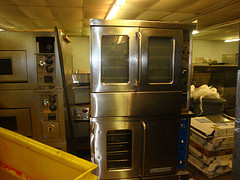The photograph captures an industrial kitchen or a warehouse filled with commercial kitchen equipment. At the center stands a prominent two-layer stainless steel oven, featuring doors with handles and clear windows on both the upper and lower levels, revealing internal shelves. To its left, another similar stainless steel oven is visible, equipped with dials and controls. In the foreground on the left side of the image, yellow plastic storage containers are seen, and a gray bin filled with used saran wrap adds to the clutter. Nearby, a stack of large white flat boxes, possibly pizza boxes, appears to the right of the ovens. In the background, additional cooking machinery and what seems to be a sink are visible. The ceiling above is paneled with lights reflecting off its surface, contributing to the overall illumination. The arrangement of these items suggests the oven might be temporarily positioned away from the wall or centered in the room, denoting this may not be its permanent location.